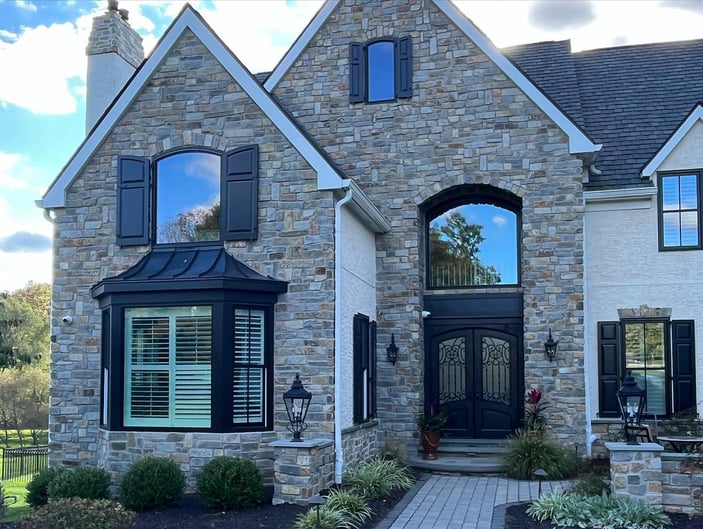The photograph captures a magnificent two-story brick home under a vibrant daytime sky, dotted with patches of blue and scattered clouds. The home's design features prominently peaked roofs and a beautiful chimney, which is also made of brick. The front façade boasts black shutters on several windows and a striking black double entry door adorned with decorative wrought iron scrollwork.

A meticulously manicured yard frames the house, with neatly trimmed bushes and colorful flowers adding to the charm. The entryway is paved and marked by elegant brick pillars on either side, each topped with a vintage-style lantern. The gray shingle roofing complements the home's classic aesthetic, while greenery from trees and shrubs surrounds the building, providing a picturesque setting.